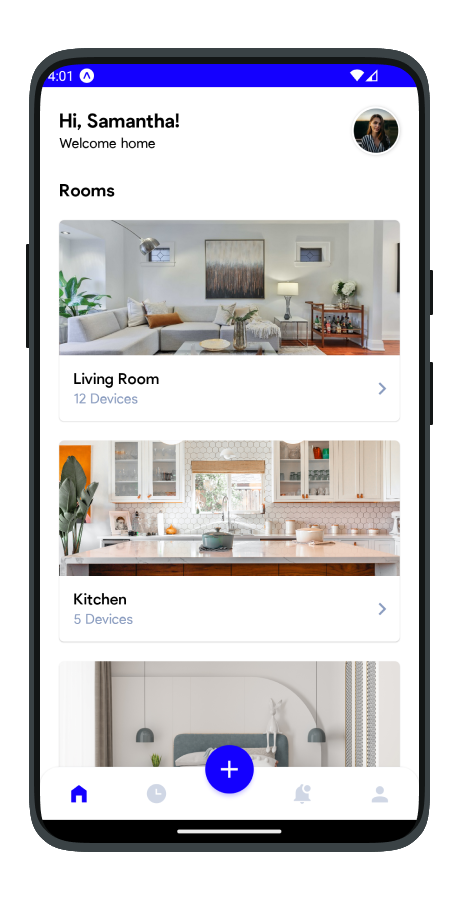The image is a high-resolution, color photograph of a mobile phone screen displaying a home control application. The phone itself has a sleek design with curved corners and a prominent, reflective silver button at the bottom center. Encasing the screen is a thin, black, curved band along the top, complementing the device's modern aesthetic.

The application interface consists of a predominantly white background with black text and features a vivid blue status bar at the top. On the left side of the blue bar, the time is displayed, showing "4:01". The right side houses a series of status icons including a white Wi-Fi symbol and signal strength bars, although the battery icon is notably absent.

Below the status bar, in bold text, is a greeting message: "Hi Samantha, welcome home." Accompanying this text on the right is a circular avatar of a woman with light skin and long hair, set against a sky backdrop. She is dressed in a grey top.

The main section of the screen is divided into two distinct parts labeled "Rooms." The first section is dedicated to a living room, depicted in grayscale with a cohesive modern design that includes a grey couch, grey walls adorned with wall art, a coffee table with a plant, a floor lamp, and a larger plant positioned on the left. The label beneath the image reads "Living Room," with an indication of "12 devices" connected.

The second section showcases a kitchen with cream or pinkish cupboards and a white countertop. A detail of note is an item hanging on an orange wall or door on the left edge of the image. This section is tagged "Kitchen," which connects to "5 devices."

At the bottom of the screen, there are additional UI elements: a grey curved surface featuring three vertical lines on the right, possibly representing a slider or separator. A centrally located blue circular icon with a white plus sign suggests the option to add new devices or rooms. To the left of the blue icon is another blue circular icon resembling a home. On the right side of the blue icon, there are three greyed-out round icons, including a generic placeholder circle, an unspecified symbol, and a profile avatar.

Overall, the application interface is clearly designed for home automation, providing a streamlined and visually coherent way to manage and monitor various smart home devices.